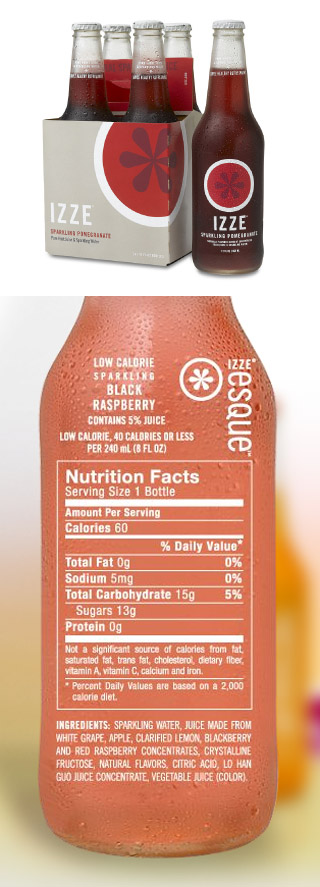Here is a detailed and cleaned-up caption for the image described:

---

The image consists of two photographs presented vertically. The top photograph features a four-pack of IZZE drinks encased in a recyclable cardboard carrier. The carrier is predominantly gray with a design that includes a red, watermelon-like circle in the corner. This four-pack holds four glass bottles filled with a dark auburn liquid. To the right side of the pack, there is an additional glass bottle placed outside the carrier, showcasing the individual bottle's design.

The bottom photograph displays a vertical image of a glass filled with an orange, almost dark orange liquid. The glass is printed with white nutritional information. Surrounding the glass are light, blurry colors in shades of lime green and orange, creating a visually appealing and vibrant background.